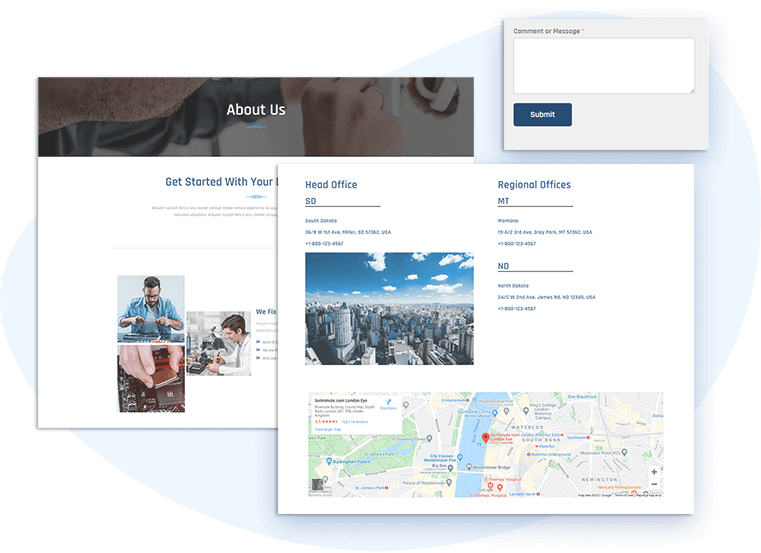The image displays three distinct web pages or pop-out sections from a web application, all arranged together against a white background. Overlaid on this background is a light blue bubble where the three elements are positioned.

In the top right corner, there is a rectangle with a gray background designated for typing a message. At the top left of this gray rectangle, the text "comment or message" is written in black, accompanied by a red asterisk. Below it is a white rectangular input field for entering a comment, with a dark blue submit button beneath that, featuring the word "Submit" in white.

The remaining part of the image consists of two large web pages, with one partially obscuring the other. The web page in the background, situated to the left, has a brown banner at the top displaying white text that reads "About Us," with a small blue line underneath. Although the right half of this page is obscured by the foreground web page, visible elements include the blue text "Get started with your" followed by unreadable text, and additional paragraph text beneath that. The page showcases three square photographs arranged in two columns. 

- The top left photograph portrays a man with dark hair, glasses, a beard, and a blue shirt over a white t-shirt, focused on an object in his hands while sitting at a table.
- Below that, there's an image of a white hand inserting a chip into a computer motherboard.
- To the right, another image shows a man in a white lab coat with dark hair and light skin, working at an electronics bench.

To the right of these photographs, the text "We fix" is visible in blue, followed by more text and three bullet points, which are cut off by the overlapping web page.

The web page in the foreground, overlapping on the right, has a white background. On the left side, a blue heading reads "Head Office, SD for South Dakota" with accompanying contact details. On the right, it lists "Regional Offices" in blue, followed by sections for "MT for Montana" and "ND for North Dakota," each with respective contact information. Further down, there's an image of a clear blue sky with white clouds over a cityscape, spanning the page's width. Beneath this image is a Google Maps snapshot displaying various labeled locations like Waterloo, South Bank, Buckingham Palace, Palace of Westminster, and Newington, suggesting a European context. The map highlights routes to a specified location, although the image is blurry and the exact details are hard to discern.